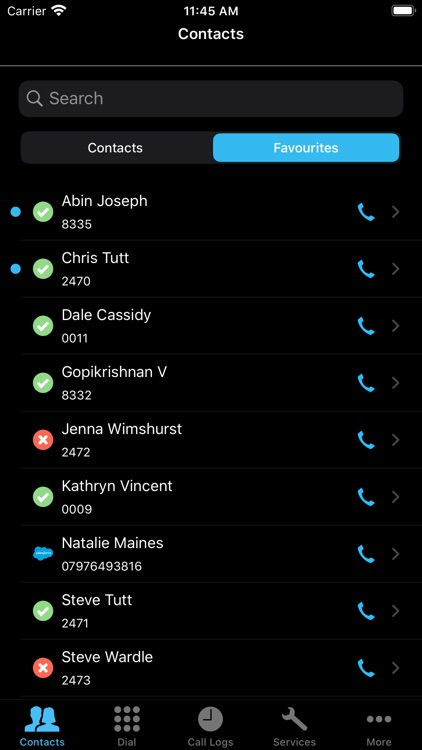This image depicts a screenshot of a smartphone's contact list interface, captured in a well-organized, user-friendly layout. 

At the very top of the screenshot, the device's status bar is prominently displayed. On the right-hand side, a fully charged battery icon is visible, represented by a white color fill. Centrally placed at the top, the current time is shown as 11:45 AM. The top left corner reads the word "carrier," accompanied by a fully connected Wi-Fi symbol.

Below the status bar, the word "Contacts" appears in white text, prominently positioned at the top. A subtle, grayish line runs horizontally beneath the title, providing a clean separation from the rest of the interface. Directly under this separator, a search bar is present, featuring the placeholder text "Search" on the left side, paired with a magnifying glass icon indicating its function.

Further down, there are two tabs for easy navigation: one labeled "Contacts" on the left, and another labeled "Favorites" on the right. The "Favorites" tab is highlighted with white text against a light blue background, indicating it is the active selection.

The main section of the screen displays a vertical list of contacts, each accompanied by a blue telephone icon on the right, signifying the option to initiate a call. The names listed are as follows: 
- Abin Joseph
- Chris Tutte
- Dale Cassidy
- GoPix V
- Jenna Wimsert
- Catherine Vincent
- Natalie Maines
- Steve Tutte
- Steve Wardle

This organized and detailed interface ensures that users can clearly navigate and make calls to their contacts with ease.